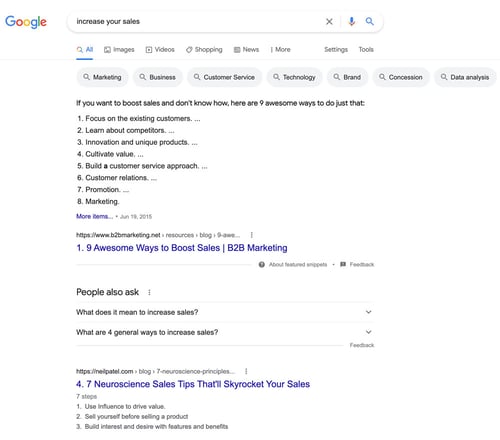The image depicts a detailed Google search results page focused on strategies to increase sales. At the top, there is a white search bar with black text that reads "increase your sales." Below the search bar, a navigation menu includes options like All, Images, Videos, Shopping, News, More, and Settings and Tools. 

Further down, there are several categorical buttons labeled Marketing, Business, Customer Service, Technology, Brand, Concession, and Data Analysis. Underneath this navigation, there is a statement: "If you want to boost sales and don't know how, here are nine awesome ways to do just that." 

Following this, the numbered list provides:
1. Focus on the existing customers
2. Learn about competitors
3. Innovation and unique products
4. Cultivate value
5. Build a customer service approach
6. Customer relations
7. Promotion
8. Marketing and further suggestions

Additionally, a link titled "Nine awesome ways to boost sales. B2B marketing" is displayed prominently. 

Further down, there is a "People also ask" section, with questions such as "What does it mean to increase sales?" and "What are four general ways to increase sales?" Each question has a downward-pointing arrow for more details. Another link in blue text reads "Seven neuroscience sales tips that'll skyrocket your sales."